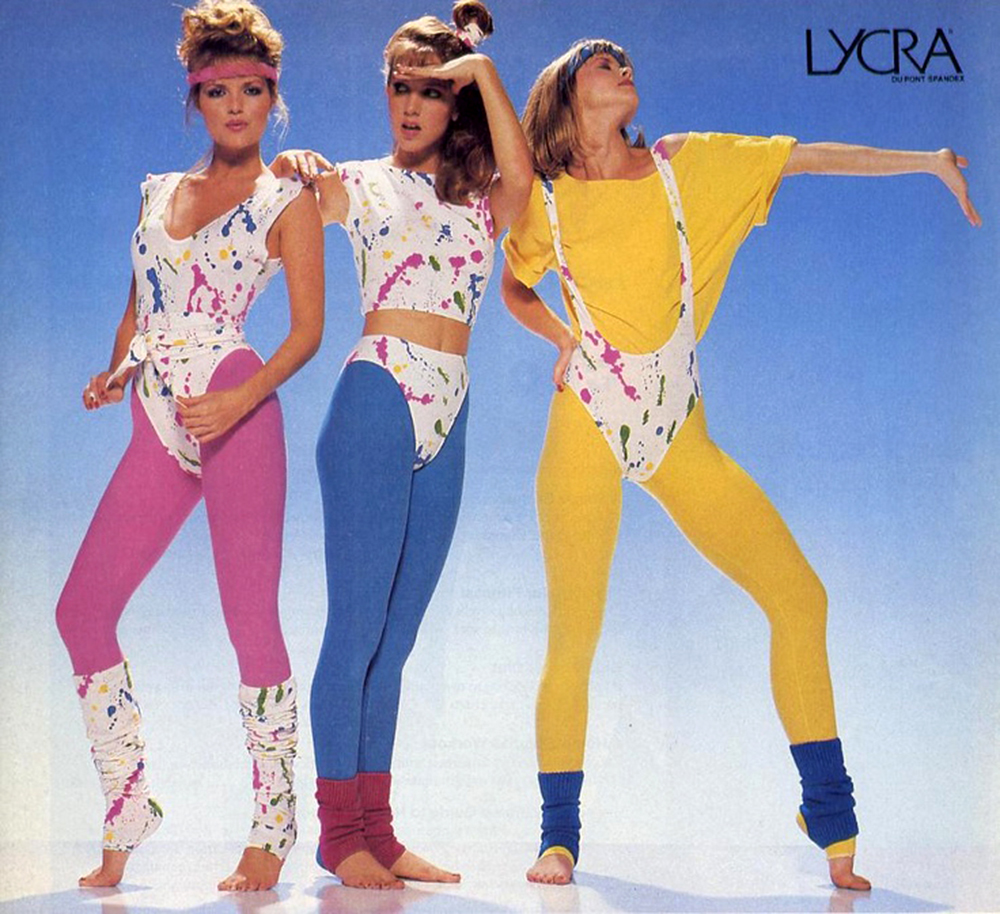This color photo is a vibrant 80s advertisement for Lyrca DuPont Spandex, featuring three young women with fair skin and brown hair striking various poses against a light blue background. The text "Lycra" and "DuPont Spandex" appears prominently in black in the upper right corner. Each woman is dressed in eye-catching, skin-tight, athletic outfits that showcase the versatility and style of spandex material.

From left to right:
- The first woman is wearing a pink sweatband and looks directly at the camera. She is dressed in a pink leotard with matching pink leggings, complemented by white tie-dye patterned leg warmers.
- The second woman stands tall with her arm resting on the shoulder of the woman next to her, and her other hand shielding her forehead as if blocking out the sun. She wears a separate white tie-dye top that shows her midriff, matching tie-dye panties, blue tights, and little red foot warmers.
- The third woman has her head tilted back, arm thrown out exuberantly. She is dressed in a scant white tie-dye top with long, thin straps, paired with a full-body yellow tights jumpsuit and blue foot warmers.

All of their outfits feature various configurations of white clothing with a vivid tie-dye pattern in pink, blue, green, and yellow, adding to the lively, dynamic feel of the advertisement. Their hair styles—ranging from up in curls, a partial ponytail, to loose long hair with headbands—further enhance the overall retro aesthetic.